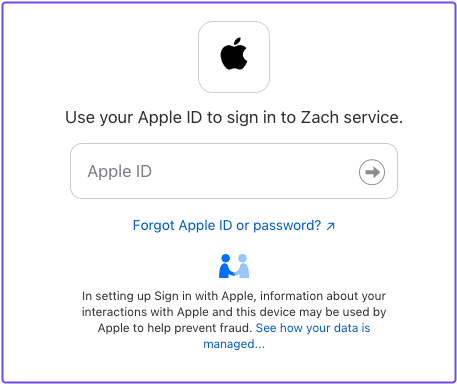This is a page on the Apple website featuring a square box centered against a white background. The square box is outlined in purple. At the top center of the box, there is the iconic Apple logo. Below the logo, the text reads, "Use your Apple ID to sign in to Zach Service."

Beneath this instruction, a text box labeled "Apple ID" invites users to enter their credentials. To the right of this text box, there's an arrow button designed to be pressed after the Apple ID is entered. Below this, a link states, "Forgot Apple ID or password," offering assistance for users who have forgotten their login information.

Further down, there are two small icons, one on the left and one on the right, depicting two people shaking hands. The text under these icons says, "In setting up sign in with Apple, information about your interactions with Apple and this device may be used by Apple to help prevent fraud." A link below this text encourages users to "See how your data is managed."

This comprehensive sign-in page allows users to access the Apple Zach Service, providing clear instructions and support options, although the specific nature of the Apple Zach Service remains unclear.